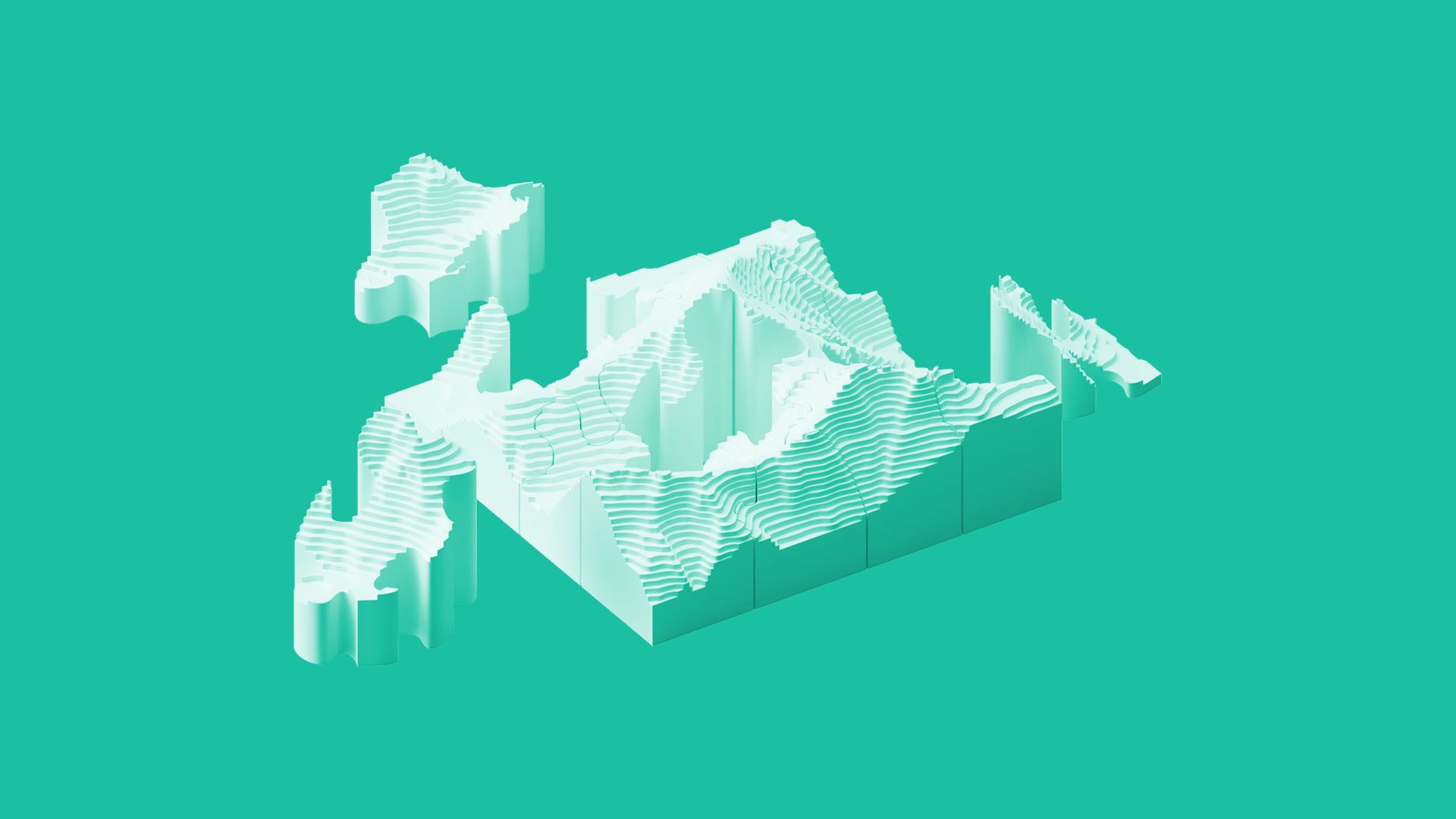The image features a horizontal, rectangular composition with a light teal-green background. Central to the composition is a large, white mass that resembles either an iceberg cross-section or a terraced landmass, similar to a 3D print due to its finely graded shapes and smooth sides. This primary structure is flanked by several smaller white chunks on both the left and right, and above, mimicking broken-off pieces of the main form. Shadows on these white elements give them a slightly bluish hue that matches the background, enhancing their three-dimensional, floating appearance. The overall impression is of a complex, detailed rendering of icy or mountainous terrain, possibly suggesting a logo or a conceptual 3D visualization used in a presentation.